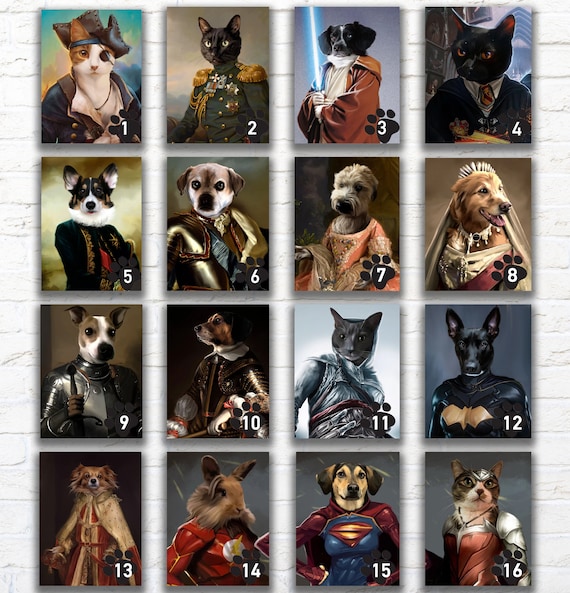The image is a grid of 16 labeled squares, arranged in four rows and columns, each separated by white bands. Each square features a portrait of a cat, dog, or small animal like a hamster, dressed in a variety of costumes ranging from medieval attire to superhero outfits. Notable examples include: a cat dressed as a pirate with a hat and eye patch; another cat resembling a general in military attire; a third cat channeling a Star Wars character with a lightsaber; and a fourth cat appearing in a Hogwarts library setting. There’s also a hamster dressed as The Flash. Each background sports different colors, such as gray, black, beige, and sky blue, adding further visual diversity to the collection.